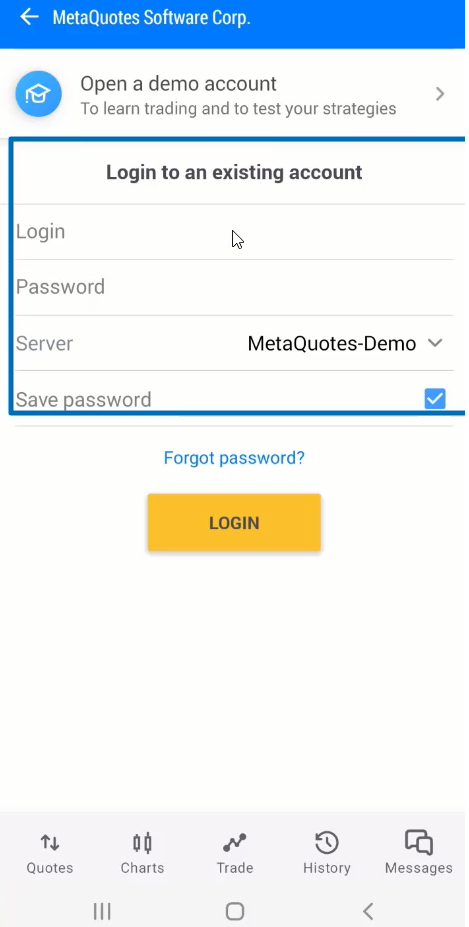Screenshot of a web window titled "MetaQuotes Software Corp." with a distinct blue header frame. The web page features a clean, white background. At the top, just below the blue frame, the text "Open a demo account to learn trading and to test your strategies" is prominently displayed. Adjacent to this text on the left is a blue graduation cap icon, symbolizing education and learning.

Beneath this informational banner is a bold and black text section labeled "Login to an existing account." This section includes fields for login credentials: a line for the username, a line for the password, and a server line labeled "MetaQuotes demo" to the right. There is also a "save password" line with a blue-checked checkbox beside it, indicating the option is selected. The entire "Login to an existing account" section is enclosed in a box with a blue outline and a white interior. Below this section, there is a "Forgot password?" link, providing assistance for users who have trouble logging in. An eye-catching orange "Login" button is prominently displayed for user engagement.

At the footer of the webpage, five icons provide quick navigation options: 

1. **Quotes** - represented by two arrows pointing in opposite directions.
2. **Charts** - depicted as two scrolls.
3. **Trade** - shown as a line graph with an upward trend.
4. **History** - symbolized by a clock with the arrow pointing backwards.
5. **Messages** - illustrated by two overlapping talk bubbles.

These icons offer users streamlined access to crucial features of the MetaQuotes platform.